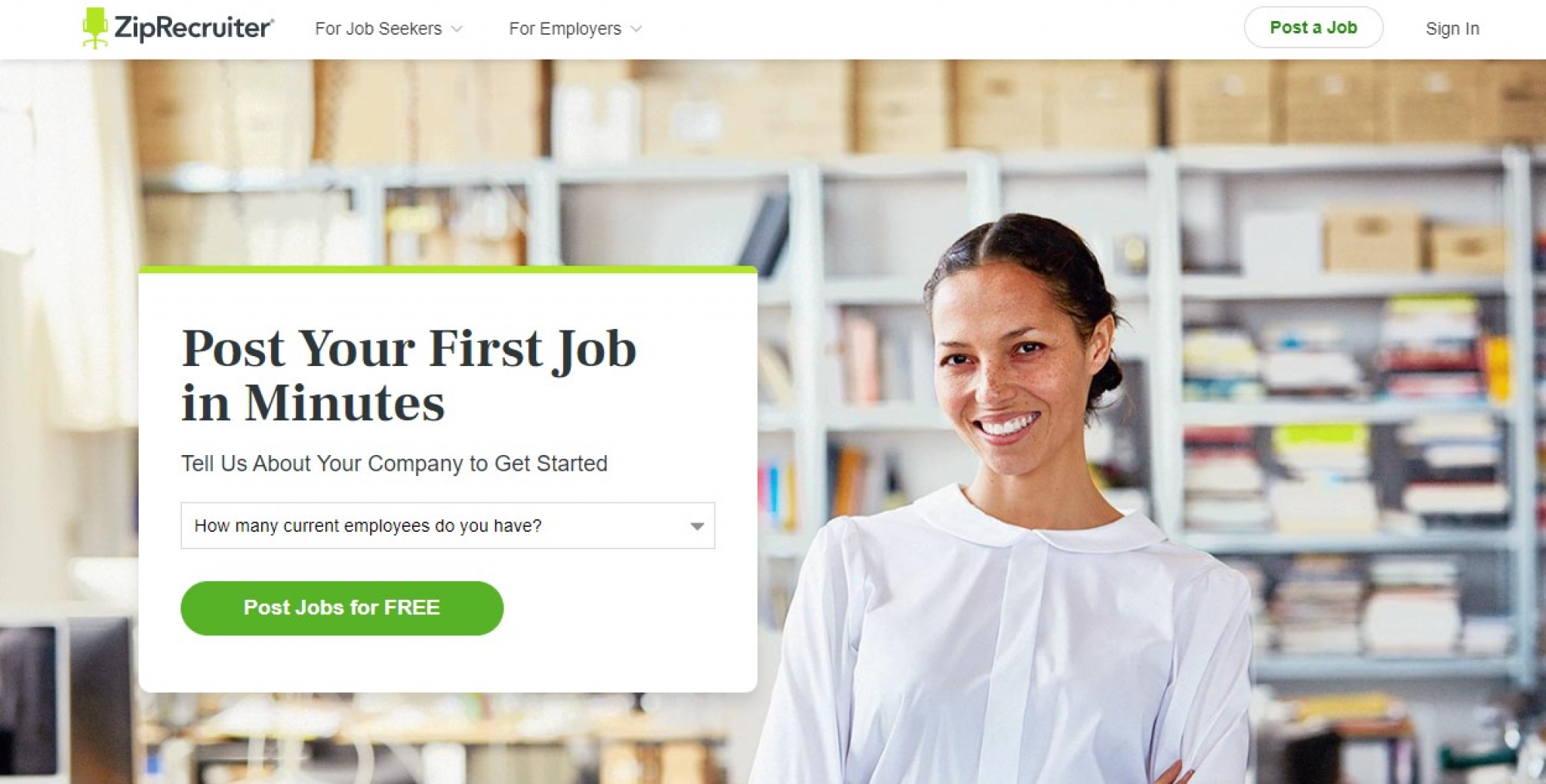This screen capture from the ZipRecruiter website serves as the landing page for employers looking to post job listings. The ZipRecruiter logo is prominently displayed in the upper left corner. The navigation bar includes options for "For Job Seekers" and "For Employers" along with buttons to "Post a Job" and "Sign In."

Dominating the center field of the image is a vibrant office setting. The background, while blurred, hints at a professional environment with shelves stocked with books and manuals. The focal point of the image is a young African American woman, likely in her mid-twenties, with a welcoming smile. She wears a white shirt, and her hair is neatly pulled back, exuding a sense of professionalism and approachability.

To the left of her, an overlay in the form of a white rectangle draws attention with the text: "Post your first job in minutes." Below this, it prompts employers with "Tell us about your company to get started." A rectangular field asks, "How many current employees do you have?" and a green oval button beneath it encourages users to "Post Jobs for Free."

This comprehensive layout efficiently guides new employers through the process of posting job listings, emphasizing ease of use and accessibility. The professional setting and the positive demeanor of the featured woman enhance the welcoming atmosphere of the site.